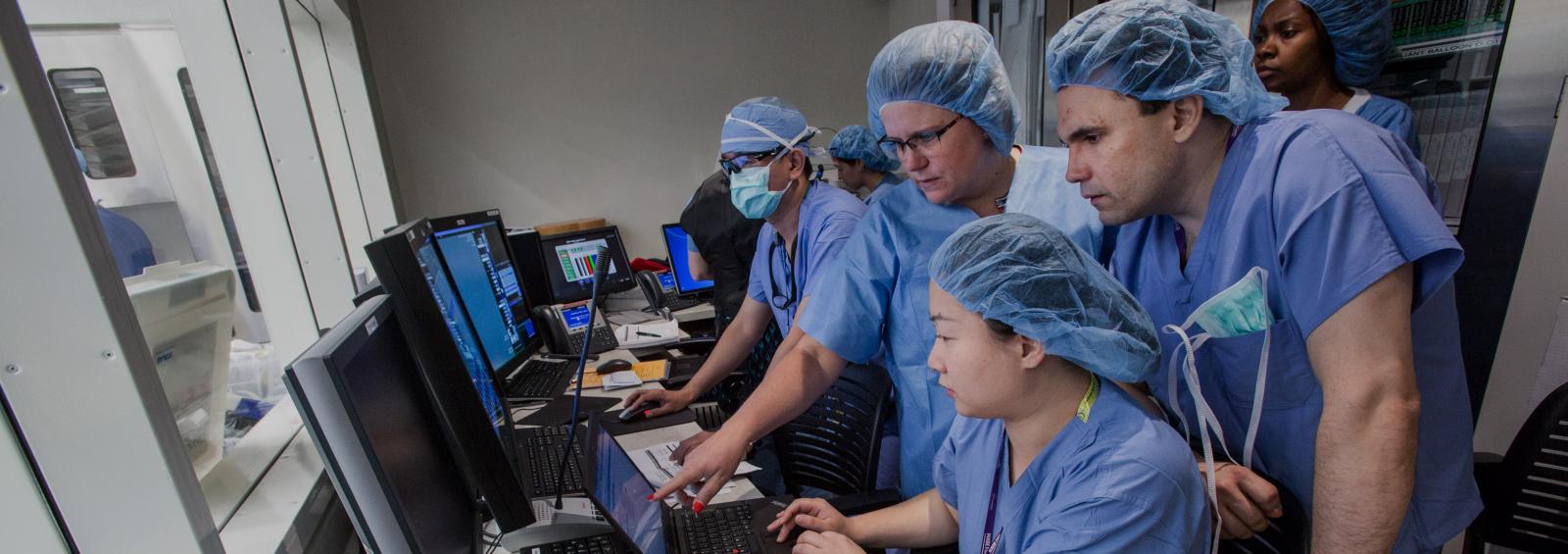This detailed photograph captures a group of doctors or surgeons intensely focused on assessing test results in a small, confined room filled with medical equipment. All individuals are wearing blue scrubs and hair nets, indicating they have likely just come from a procedure. Among them, one doctor is wearing a mask and what appears to be protective goggles, further emphasizing the serious nature of their work. The group includes diverse racial backgrounds: an Asian woman typing on a keyboard, a Caucasian man directly behind her, a black medical professional standing nearby, and another Caucasian woman with bright red fingernails. They are clustered around several screens—at least five or six—arranged on a table cluttered with laptops, phones, and various work-related items. One of the doctors is pointing at a screen, indicative of a serious discussion, while large windows behind them reveal a faint glimpse of a person in an adjoining room, suggesting an ongoing medical procedure. The overall atmosphere is one of intense concentration and teamwork.